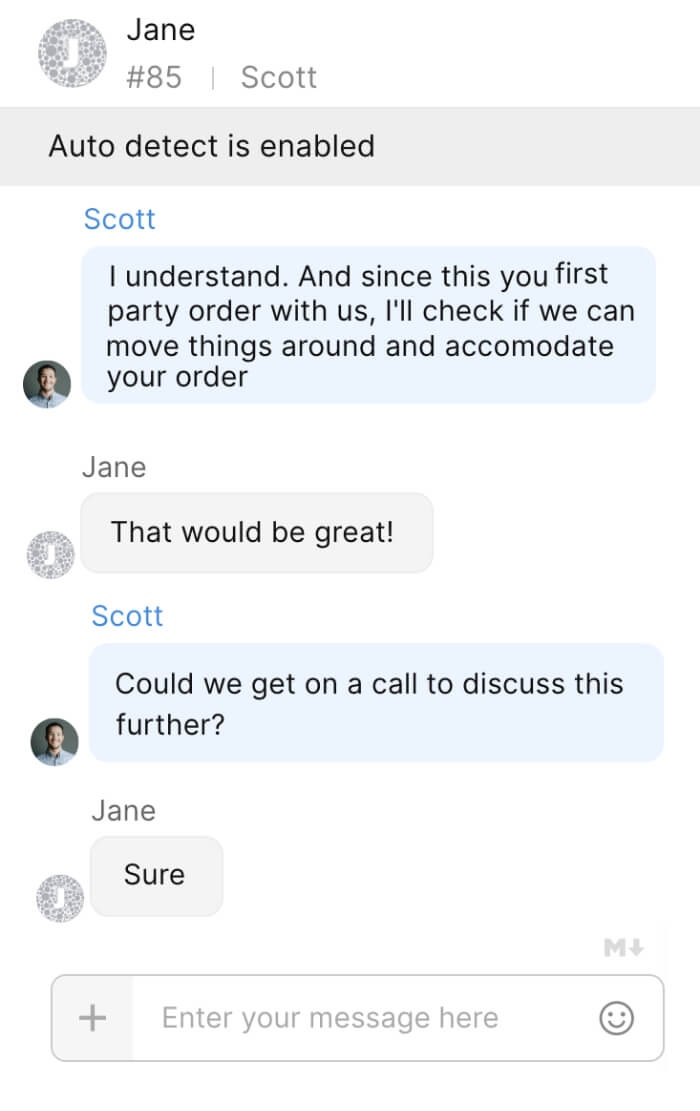The image is a screenshot of a series of text messages displayed on a smartphone. At the top of the screen, there is a circular icon with a white 'J' inside, surrounded by smaller gray circles, indicating contact initials and possible message threads. To the right, the contact name "Jane" is displayed, with an identifier "85, Scott" listed below it. 

Beneath the contact information, there is a long, gray rectangle with black text that reads "Auto detect is enabled." Following this, "Scott" is highlighted in blue, accompanied by an icon showing a photograph of a male. In a light blue conversation bubble, Scott's message reads, "I understand, and since this is your first party order with us, I'll check if we can move things around and accommodate your order."

Below Scott's message, Jane replies in a gray-colored text bubble, stating, "That would be great." Scott then responds in another light blue bubble, "Could we get on a call to discuss this further?" Jane answers in a gray bubble with a single word, "Sure."

At the very bottom of the screenshot, there is a narrow rectangle featuring a plus sign to the left. This field is intended for inputting a new message and is labeled "Enter your message here." A smiley face icon is positioned to the right of this input field.